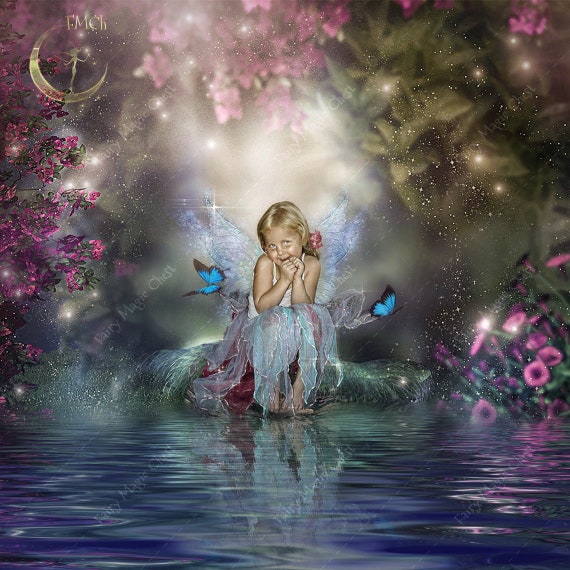This detailed digital drawing features a young girl, approximately 3 to 5 years old, seated on a glittering rock near a blue body of water. With her hands held close to her chin in a delightful, almost shy smile, she exudes an enchanting charm. She has light blonde hair pulled back into a ponytail adorned with pink flowers. Clad in a translucent, glittery fairy costume, her attire, comprising a long, flowing skirt that shimmers in hues of turquoise, green, and white, complements her ethereal appearance.

The fairy wings on her back glow brilliantly, appearing transparent with a hint of blue glitter that adds a magical touch. Surrounding her are two butterflies, their wings a striking shade of turquoise blue with black tips, fluttering gracefully. The water beneath her catches and reflects the ambient light, creating ripples laced with shades of pink.

Around her, a vibrant fairy world comes to life with glowing pink and green flowers dusted with fairy sparkles. The background is filled with various shapes reminiscent of plants, stars, glitter, and light, creating a vivid and otherworldly scene. Amidst this lush surrounding, a bed of green moss or leaves seems to support her, adding to the natural, enchanted atmosphere.

In the top left corner is a subtle, golden crescent moon logo with a small, human-like figure delicately balanced on it, adding a touch of whimsy and fantasy to the piece. The image is suffused with a magical glow, blending stars and sparkles, which enhances the dreamlike quality of this enchanting artwork.